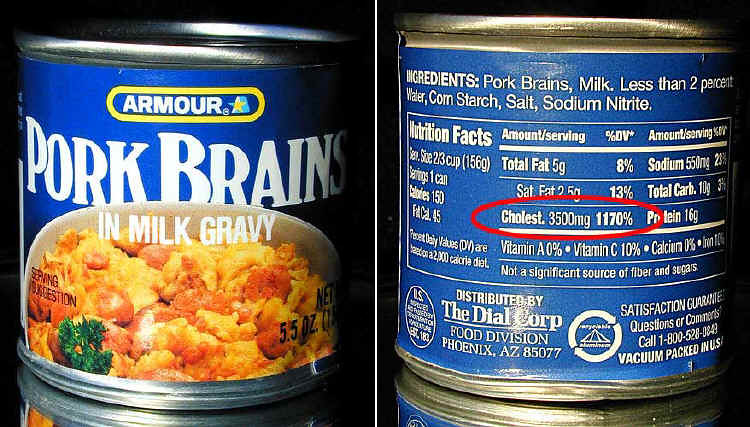The image features two photographs placed side-by-side with a thin white line separating them. The photo on the left shows the front side of a tin can labeled "Pork Brains in Milk Gravy," complete with a wrap-around label. The label includes an image of a white bowl containing the pork brains and gravy. The photograph on the right showcases the back side of the same tin can, specifically highlighting the nutrition facts. Notably, a red circle draws attention to the can’s cholesterol content, which is striking at 3,500 milligrams, equating to 1,170% of your daily recommended value.